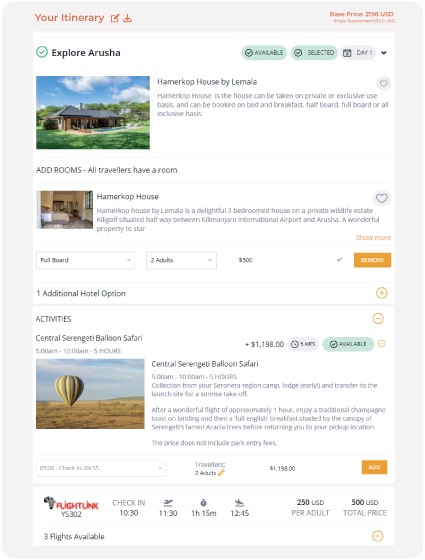**Caption:**

The itinerary showcases an exciting adventure beginning in Arusha, with accommodations at the luxurious Hammerkop House by Lamala. This exclusive residence can be reserved on a private basis and offers flexible meal plans including bed and breakfast, half board, and full board options. 

The highlight of the trip includes a breathtaking Central Serengeti Balloon Safari, promising an aerial view of the stunning Serengeti landscape. Despite the slightly clumsy translation of the app, the plans reveal a full board stay for two adults, with an all-inclusive package total exceeding $2,000. The itinerary notes the balloon flight check-in at 10:30 local time, ensuring a well-organized start to this unforgettable journey.